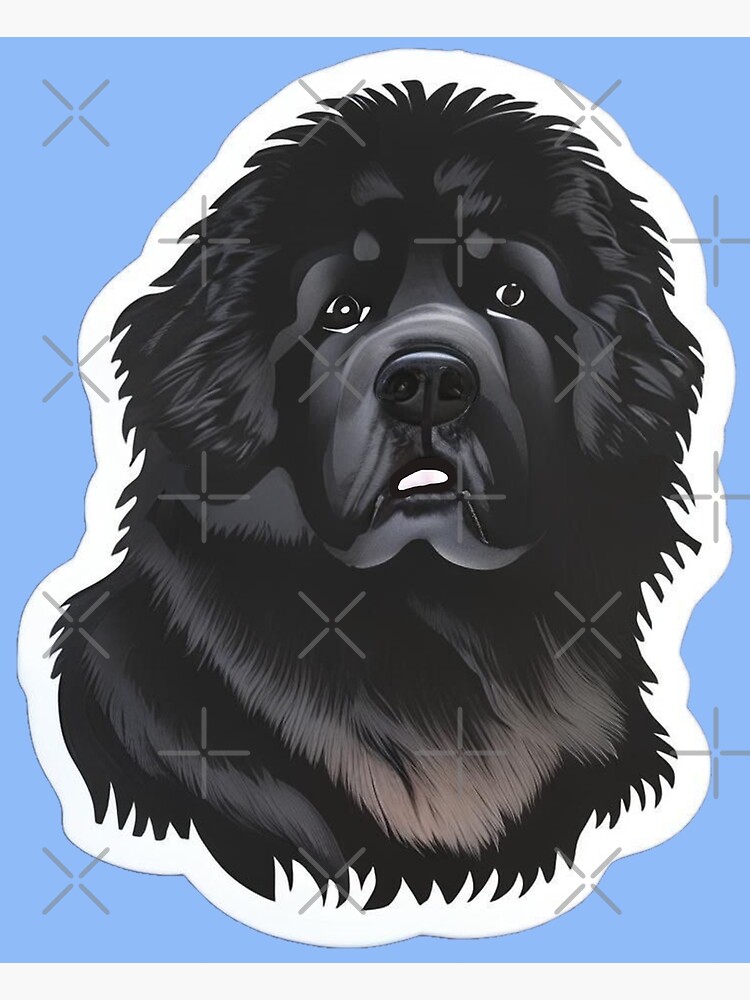The image features a cartoon-style sticker of a fluffy, black dog, possibly resembling a Labrador, Great Pyrenees, or Burmese breed. The dog's fur includes gray and brown accents around the chest, and it has notable white markings: outlines around the eyes, a white mouth, and a white streak on the nose. Its ears are down, contributing to its somewhat concerned expression. The sticker prominently displays the dog's head and upper chest, all encased within a white border. The background of the image is a light blue, overlaid with subtle watermarks in the form of X's and plus signs, serving as a protective measure against image theft.